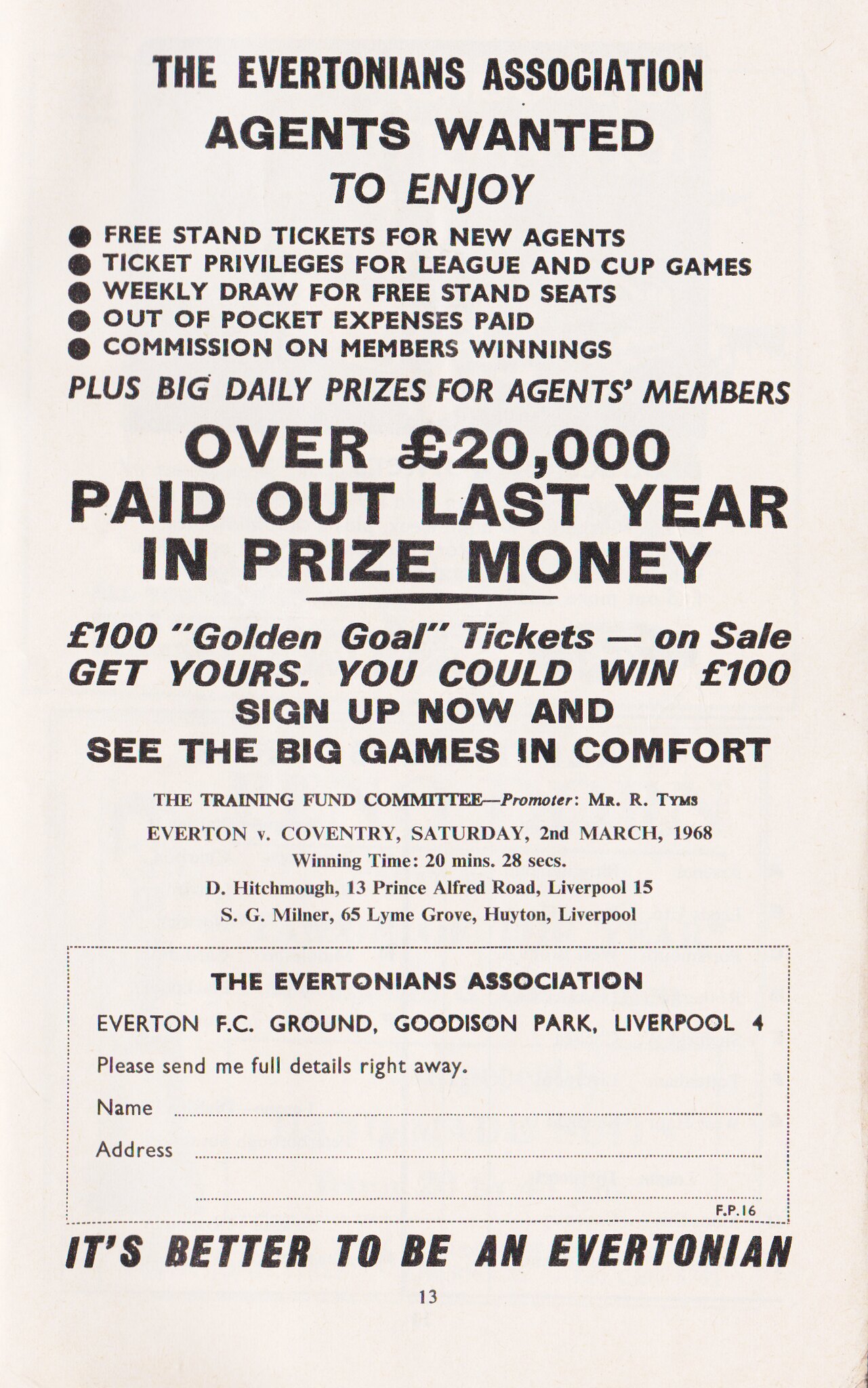The flyer for the Evertonians Association prominently features a bold heading that reads "Agents Wanted." Underneath, it lists five bullet points detailing the perks available to agents: free stand tickets for new agents, ticket privileges for League and Cup games, weekly draws, out-of-pocket expenses paid, and commission on members' winnings. The flyer emphasizes a significant opportunity, stating in large letters that over £20,000 was paid out last year in prize money. Below this, it highlights an enticing offer of £100 Golden Goal tickets on sale with the chance to win £100. The flyer encourages immediate action with "Sign up now and see the big games in comfort." At the bottom, there is a sign-up area for name and address, accompanied by the tagline, "It's better to be an Evertonian." The flyer is printed in black text on off-white paper, with key information and headings in bold and large font for emphasis.